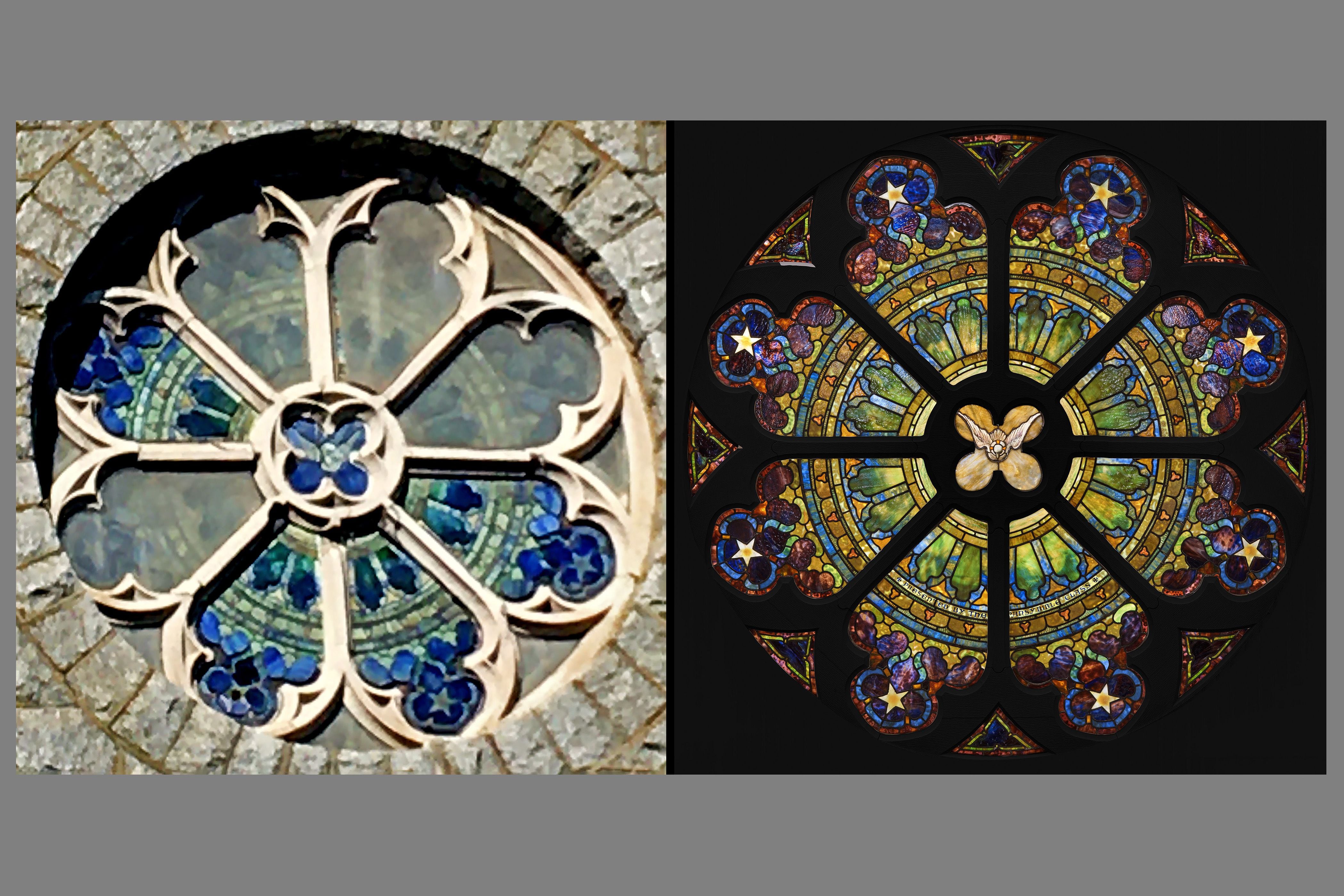The composite image features two side-by-side square pictures of the same circular stained glass window, set against a gray background. The window design resembles a flower, with a central circle surrounded by eight petal shapes. The left image shows the exterior view of the window, framed by a circular brick archway. The stained glass, partially damaged, is missing some panels, leaving empty petal frames. Some remaining panels display a blue and green ornate design. The right image renders a complete and vibrant version of the stained glass as it would appear restored. This view likely captures the interior perspective, showing a full spectrum of colors including purples, greens, yellows, and beige, arranged in a star-shaped, mandala-like floral pattern. The daytime lighting accentuates the vivid blues prominently, while at night, the other colors—purples, greens, yellows, and beige—stand out more against the dark background, creating a striking contrast with the brick frame almost blending into the night.